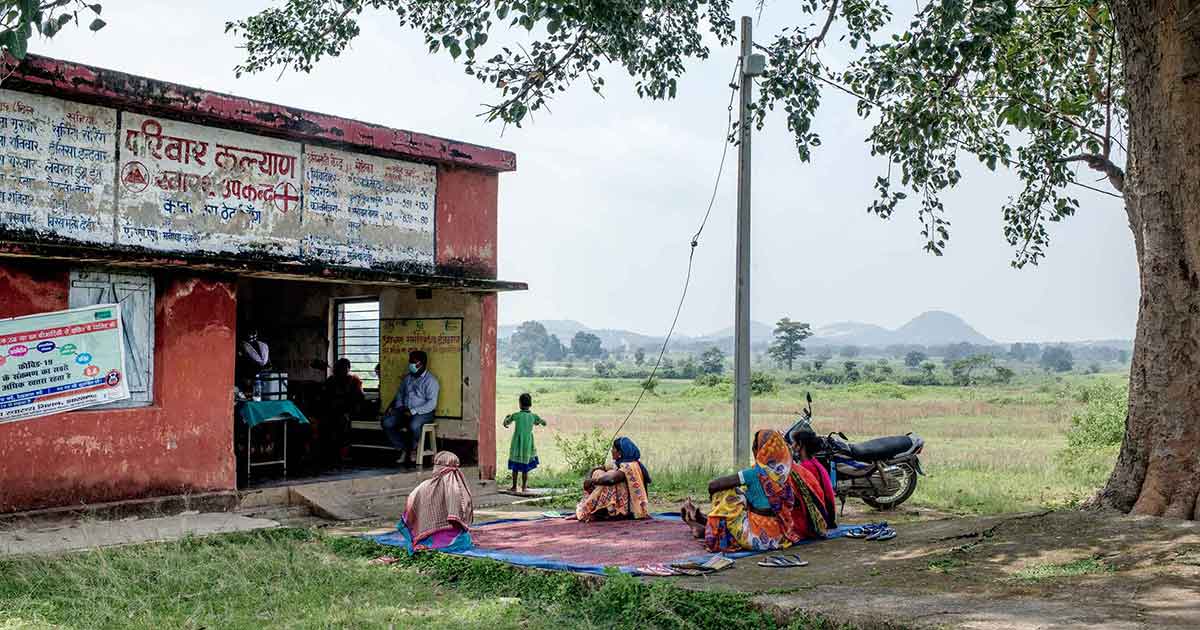This photograph depicts a rural Indian scene set in the daytime, showcasing a pink-walled store or establishment with extensive but faded writing in red and blue at the top. The structure, characterized by a wide, doorless opening, possibly features a retractable sliding door, facilitating easy access. In front of the entrance, four women adorned in head garments and long dresses are seated on a pink mat, having removed their shoes. A child accompanies them, positioned between the women and the store. Inside the building, a man sits on a bench, dressed in a long-sleeved blue shirt and denim jeans with a mask on his face, indicating the COVID-19 era. To the right of the women, a prominent tree and a tall pole with wiring are noticeable. Behind the tree, a black motorcycle is parked. The backdrop showcases a verdant landscape with a large grassy field, some areas of dried grass, and distant mountains.